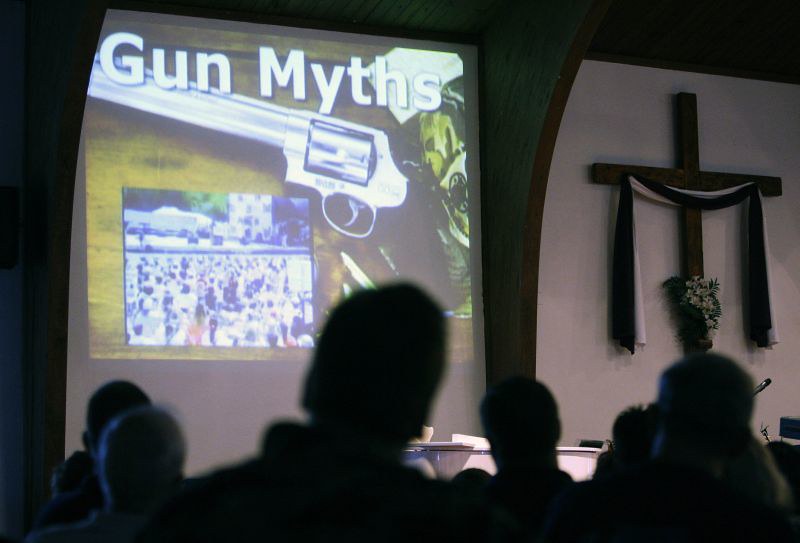This detailed image captures an interior scene of a church during a presentation on "Gun Myths." Dominating the right side of the image is a white-painted back wall adorned with a dark brown wooden cross. Draped across the cross is a black and white scarf, creating a striking contrast. At the base of the cross lies a white floral bouquet, adding a delicate touch to the somber setting. On the left side, a projection screen displays a large revolver with the white text "Gun Myths" prominently above it. Below the revolver, the projection shows a crowded scene, although specific details are obscured by darkness. In the foreground, the dim lighting reveals the silhouettes and shadows of multiple seated individuals, suggesting an attentive audience engrossed in the presentation. The overall ambiance is one of solemn reflection and attentiveness within a sacred space, as the congregation appears to engage with the content presented on the screen.